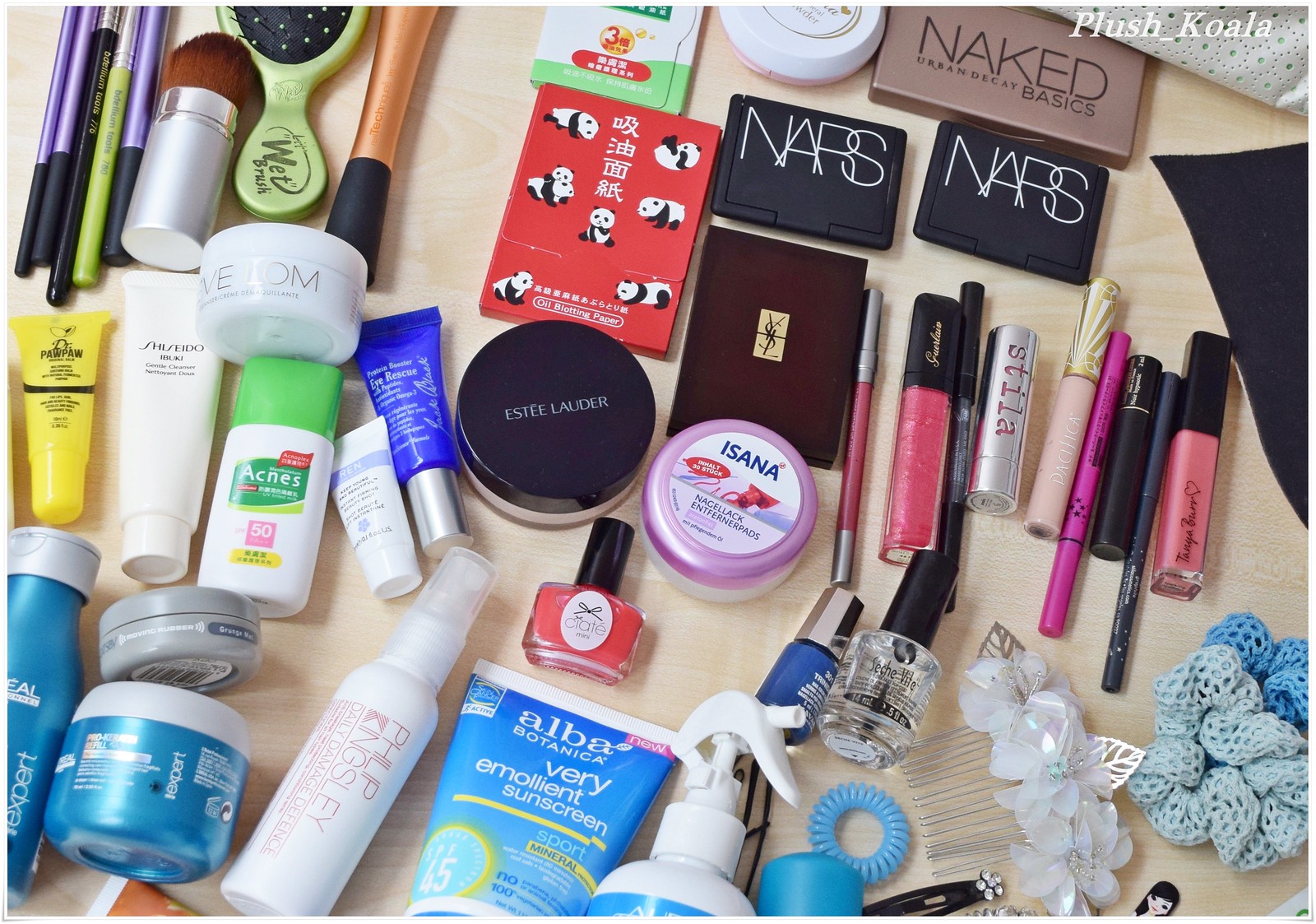The image showcases a detailed assortment of beauty supplies and hygiene care products. In the top-right corner, the name "plush_koala" is visible, indicating the owner or brand associated with the collection.

Starting from the top left, several eyeliner pens, predominantly purple with black caps, are neatly arranged. Next to them is a green brush with a black handle, as well as a green hairbrush featuring a black center and black bristles tipped with green dots. A silver-handled brush with brown bristles is also present.

In the central area, various tubes of creams and lotions in yellow, white, and blue are positioned. The left-hand side contains more containers, which are blue and silver, along with a white spray bottle embellished with pink writing.

On the right side of the image, there is a large collection of lip glosses and lipsticks, accompanied by black boxes labeled "NARS" and a "Naked Urban Decay Basics" box. Additionally, a red matchbook-shaped item with red, white, and black handles is present.

Towards the bottom of the image, several hair scrunchies, hairpins, and nail polish bottles, including a clear one and some colored options, are displayed. A large white spray bottle with a blue label is situated at the bottom, accompanied by various hair clips on the bottom right side.

The array of products covers a wide range of beauty and hygiene needs, meticulously arranged to showcase their variety and purpose.